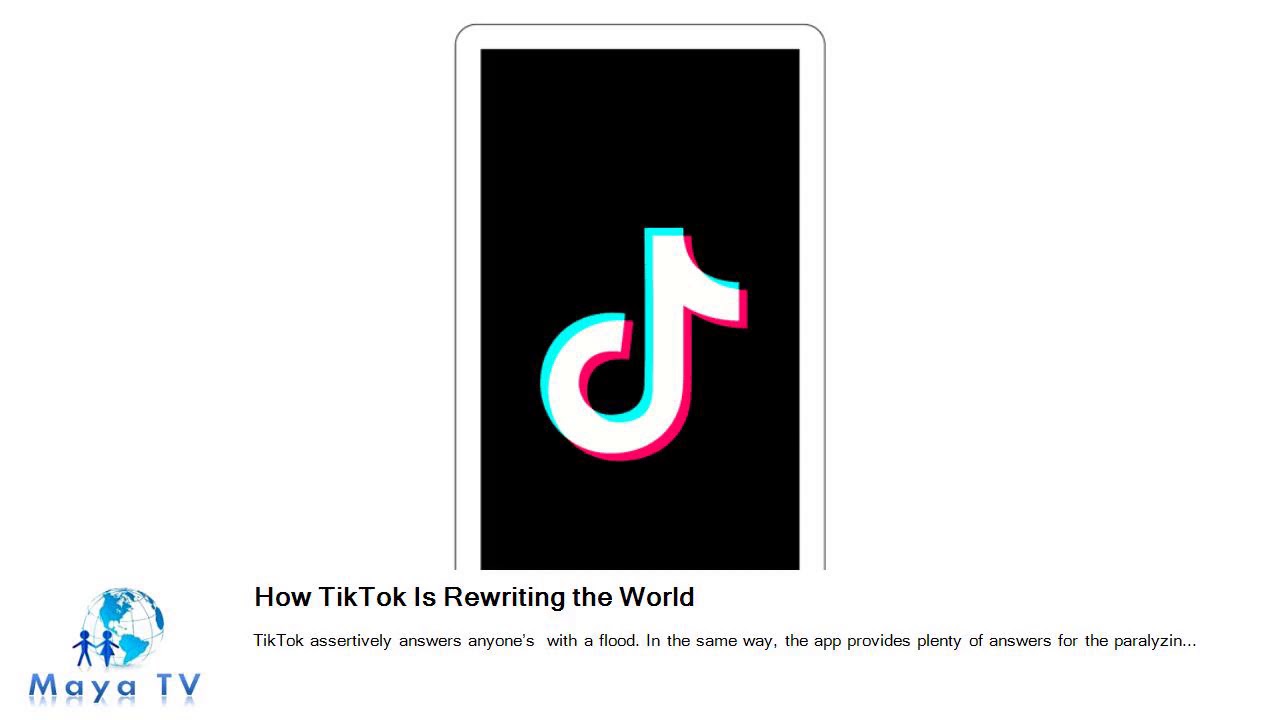An image resembling a smartphone screen displaying a TikTok interface dominates the rectangular frame, which features rounded edges and a white border. The center is filled with a black background that transitions into a square, angular space with pronounced, pointy corners, creating a stark contrast. 

In the center, the iconic thick white TikTok music note symbol takes prominence. The left side of the music note is outlined with a light aqua border that elegantly curves around to the left. On the right side, the music note is bordered by a dark pink hue that extends slightly beneath the lower curve of the note.

In the bottom left corner, a globe icon is situated next to two blue stick figure silhouettes holding hands— one figure appears in a skirt (suggesting a female) while the other figure seems to be in pants (indicating a male). Below these figures, the text "Maya TV" is boldly spaced out, with the "M," "T," and "V" capitalized.

Directly beneath the phone-shaped icon, a headline in black reads, "How TikTok is rewriting the world." Under this headline, it continues in smaller black font with the text, "TikTok assertively answers anyone's...". The sentence remains incomplete, trailing off with a flood period, and the passage continues further down with "...the app provides plenty of answers for the paralyzing...", which also cuts off with an ellipsis. The lower portion of the imaginary phone appears truncated to accommodate the placement of the headline text.